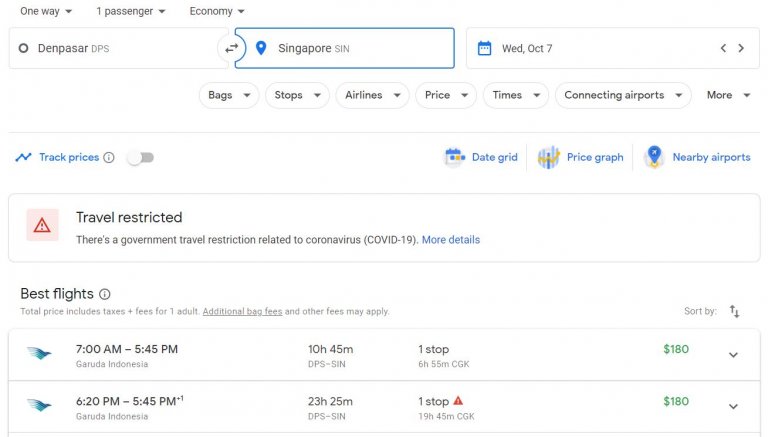This image is a screenshot of a travel booking interface. 

At the top left, there is a navigational header displaying trip details: "One Way," "One Passenger," and "Economy," each accompanied by a small downward-pointing arrow, portrayed in gray text. 

Beneath this header, three distinct input boxes are visible. The first box is labeled "DENPASAR (DPS)," the second one is labeled "Singapore (SIN)," and the third box indicates the date: "Wednesday, October 7th."

Below these boxes, there's a row of options presented as oval buttons. These options include "Bags," "Stops," "Airlines," "Price," "Times," "Connecting Airports," and "More," each with a downward arrow for additional filtering.

Further down, a section in blue text offers various features: "Track Prices," "Date Grid," "Price Graph," and "Nearby Airports," each accompanied by a relevant icon.

A prominent notification in larger black text reads "Travel Restricted," informing users of a government travel restriction related to the coronavirus (COVID-19).

At the bottom, the "Best Flights" section is displayed, showing two different flight options, both priced at $180.